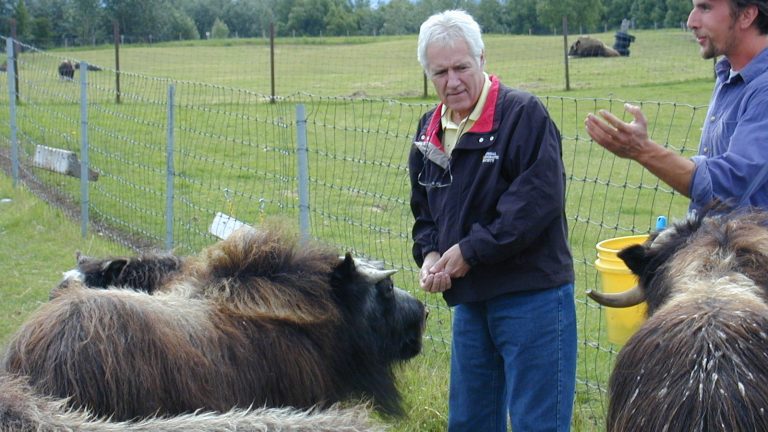In the photo, two men stand in a lush, green field facing a pair of fur-covered animals, which resemble yaks with their long, tan and brown fur and prominent horns. The man on the left, possibly resembling Alex Trebek, has receding white hair and is dressed in a black jacket with a red interior, along with blue jeans. He appears to be holding food, seemingly to feed the animals. A yellow bucket is visible near his feet. To his right is another man wearing a light blue button-up shirt with the sleeves rolled up to his elbows. He is mid-conversation, his hand raised as if gesturing to the man in the jacket.

Behind them, a chicken wire fence supported by silver metal poles delineates the immediate area, while a second fence of similar construction stands further back, this time with brown poles. The expansive green field stretches out to a horizon marked by a tree line with leaves in full bloom. Scattered around the field and near the fenced area are additional animals, adding to the pastoral scene under the bright daylight.